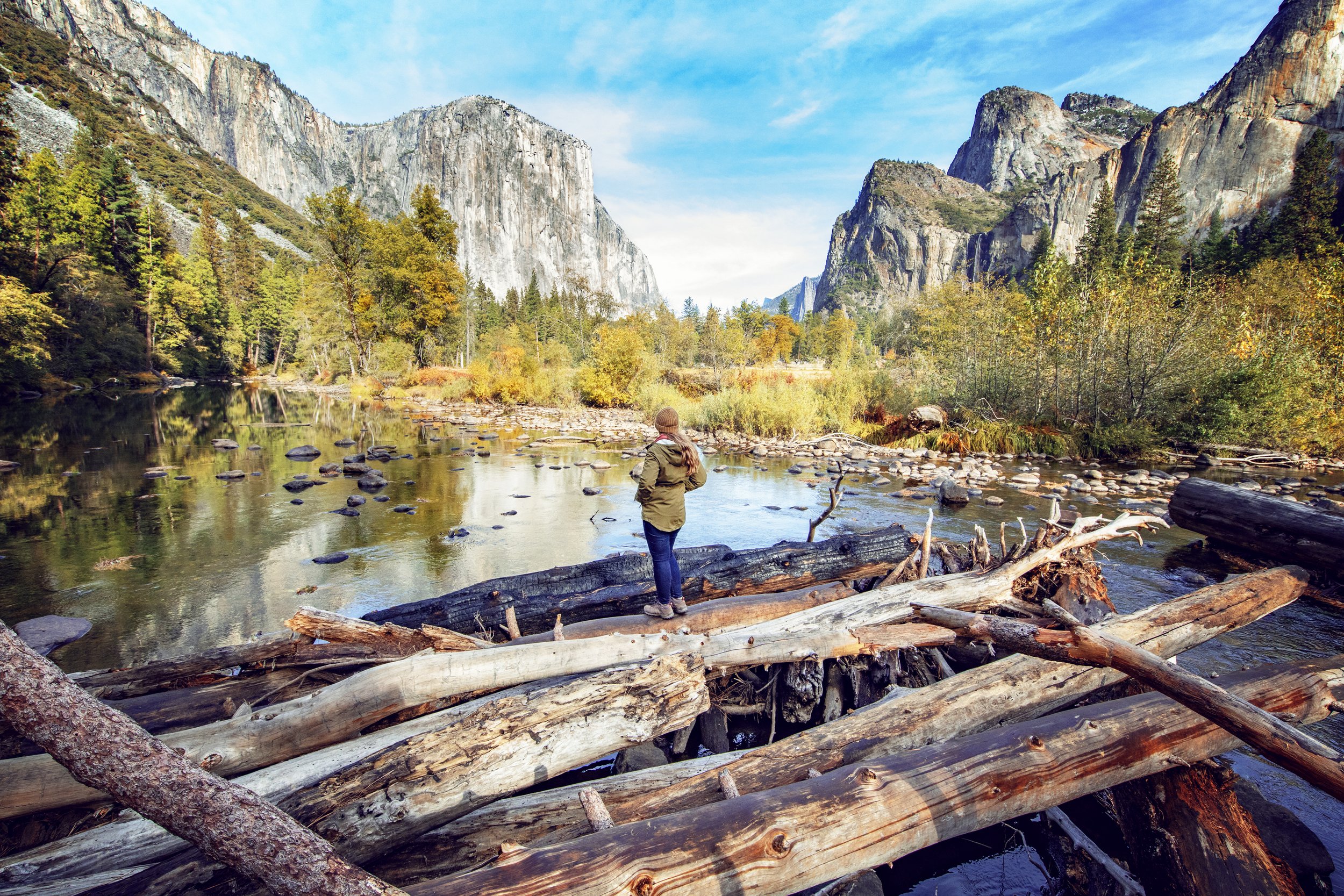In this vibrant outdoor photograph, a woman stands with her back to the camera, gazing into the horizon from atop a large, makeshift log dam. She is dressed in an olive green jacket, blue jeans, and brown boots, with long blonde hair flowing beneath a brown hat. The dark brown and white logs beneath her are floating in a body of water, possibly a river or a small lake, that runs through a valley framed by towering stone mountains on either side. 

The photo captures the interplay of nature's elements, showcasing a backdrop of lush green trees that transitions into the rocky mountains. The scene is bathed in sunlight, with a bright blue sky featuring a few scattered clouds. Pebbles and rocks are visible in the clear water below, enhancing the natural, serene atmosphere. The foliage hints at the beginning of fall with some leaves turning brownish-orange, while evergreens add splashes of deep green throughout the landscape, making for a stunning and tranquil composition.